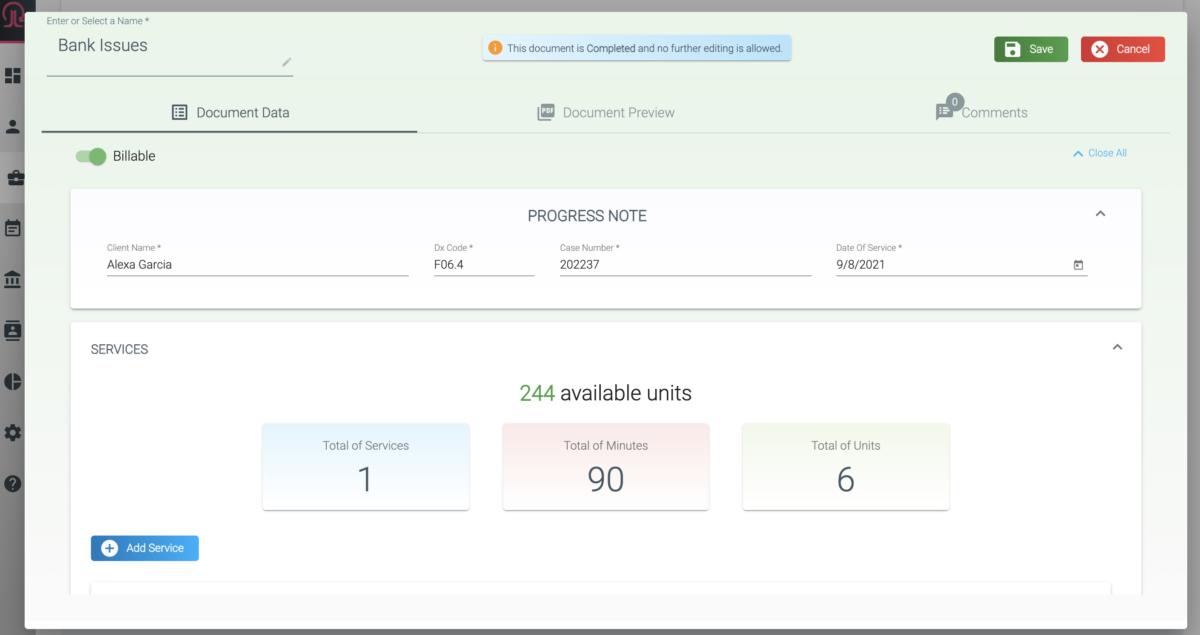The image is a detailed screenshot related to banking information. It features a gray background with visible elements of a computer interface on the left side. Overlaid on this background is a large, light green rectangle that transitions into white at the bottom.

In the upper left-hand corner of this rectangle, the title "Bank Issues" is displayed. The interface contains three tabs: "Document Data," "Document Preview," and "Comments," with "Document Data" currently selected. Below this, there is a toggle switch labeled "Billable."

The content within the rectangle includes a white section titled "Progress Note," which lists details such as Client Name (Alexa Garcia), DX Code, Case Number, and Date of Service (9-8-2021). Below this section is a "Services" rectangle showing 244 available units and three sub-sections in pastel gradient boxes:

- "Total of services" in blue: 1
- "Total of minutes" in coral: 90
- "Total of units" in light green: 6

A "Add Service" button in blue is also present, suggesting the option to include additional services.

This screenshot likely represents a pop-up screen on a financial website, possibly related to managing or reporting a financial transaction, order, or money transfer, and highlights a specific banking issue.